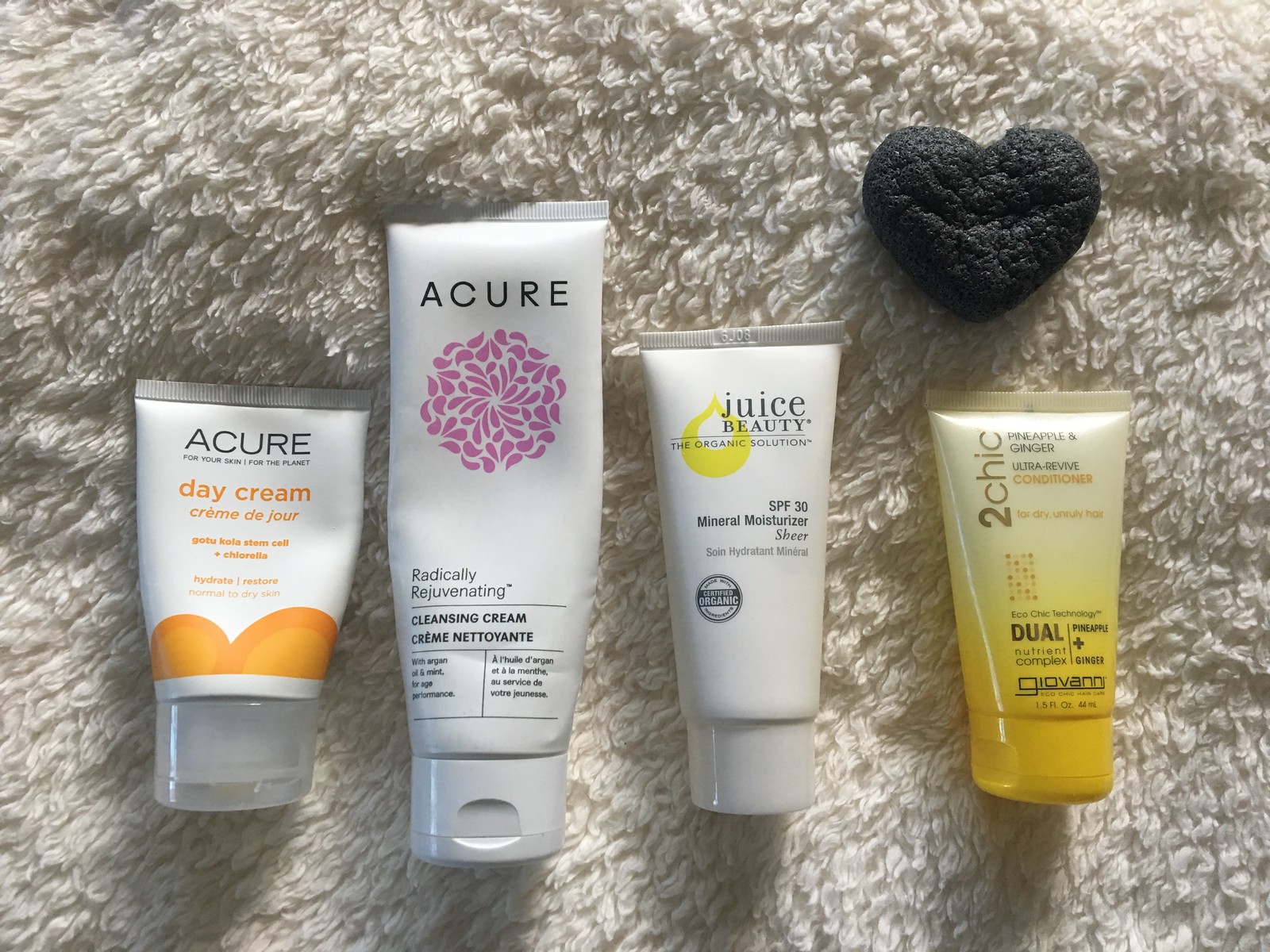In this photograph, four skincare products are meticulously arranged in a straight line on a plush, white, and fluffy surface that resembles a bath mat or cozy blanket. Starting from the left, the first product is a white bottle with its cap oriented downwards. The brand name "Acure" is prominently displayed in black lettering, with "Day Cream, Crème de Jour" written in orange beneath it. An orange circular design adorns the lower part of the bottle, near the cap.

Beside it is a slightly larger bottle, also from Acure and similarly positioned with the cap facing downward. This bottle features a dense cluster of pink flower petals just below the brand name, with the label "Radically Rejuvenating Cleansing Cream" written beneath the floral design.

The third item in the lineup is a smaller bottle labeled at the top with "Juice Beauty." It is also cap-down and includes a black circular stamp indicating that the product is "Certified Organic."

The fourth and smallest bottle in the row is yellow, transitioning from a lighter shade at the top to a darker shade at the bottom near the cap. It is labeled "Too Chic," along with "Pineapple and Ginger Ultra Revive Conditioner."

Above this final bottle rests a heart-shaped black item, possibly an exfoliating scrub or some other skincare accessory, adding an intriguing element to this orderly display.